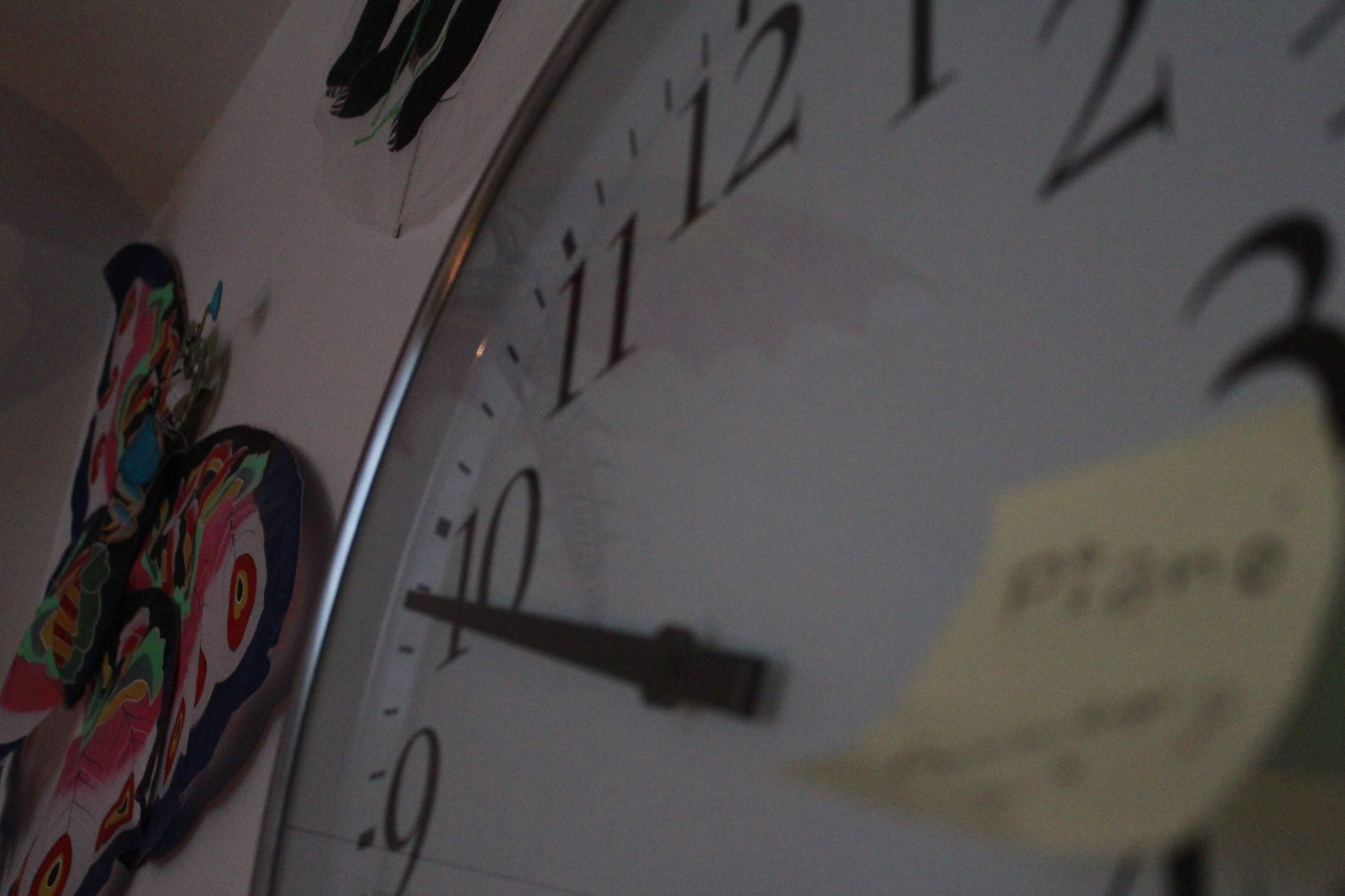This extreme close-up image showcases a clock hanging on a wall, photographed from a unique angle that provides an intimate view of the numbers. The camera is positioned at the number three on the clock, capturing a perspective that looks towards the number 10, which sits on the left side of the frame. The image cuts off the top and bottom portions of the clock, revealing only the very tip of the number four. Prominently featured next is the number nine, which is fully visible. The clock is mounted on a wall painted in a soft whitish-pink hue. Adding a touch of whimsy to the scene, there is a delicately crafted butterfly made from paper affixed to the wall.